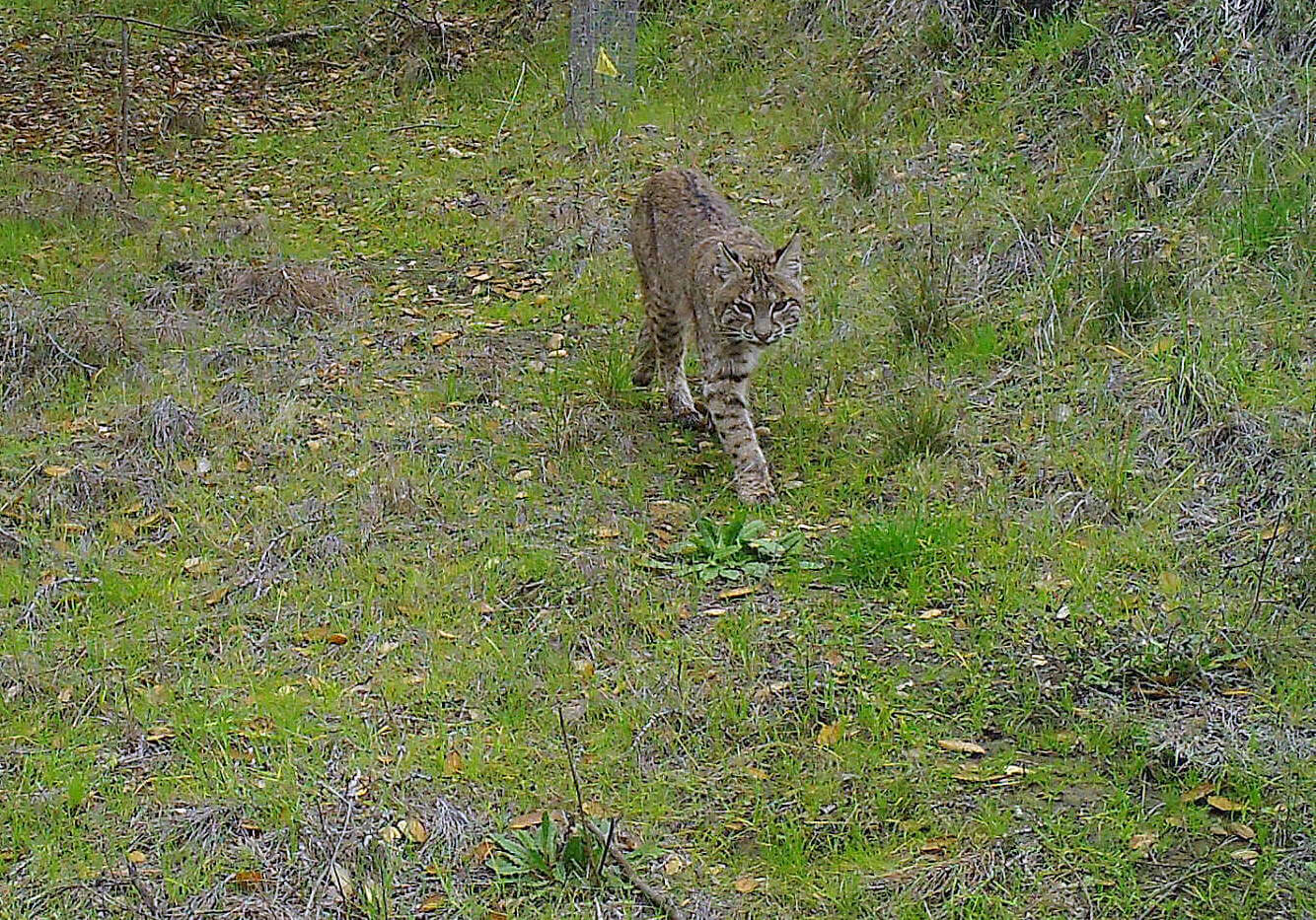The image depicts an outdoor scene captured during the daytime, featuring a bobcat, although it has some characteristics that could make it confused for a lynx. This wild feline, larger than a typical house cat, stands out in the center of the photo, walking towards the camera. The bobcat's fur is a mix of gray, light brown, and black, with noticeable spots and stripes. Its face, adorned with black stripes and white outlines around its eyes and nose, exhibits a keen and instinctive look, possibly not yet noticing the camera. The cat's dark eyes and pointed ears add to its striking presence.

The setting is a grassy clearing with unmanicured, freely growing grass, mixed with brown patches of dead plants, small yellow leaves, and various weeds. Sticks and pieces of wood are scattered throughout. The grass ranges from muted green to vibrant green shades. A notable yellow flag in the background accentuates the colors in the scene, which also include some blacks and whites. The overall ambiance of the image suggests that it could be an amateur photograph or one taken by a wildlife camera, capturing the essence of the bobcat in its natural habitat.